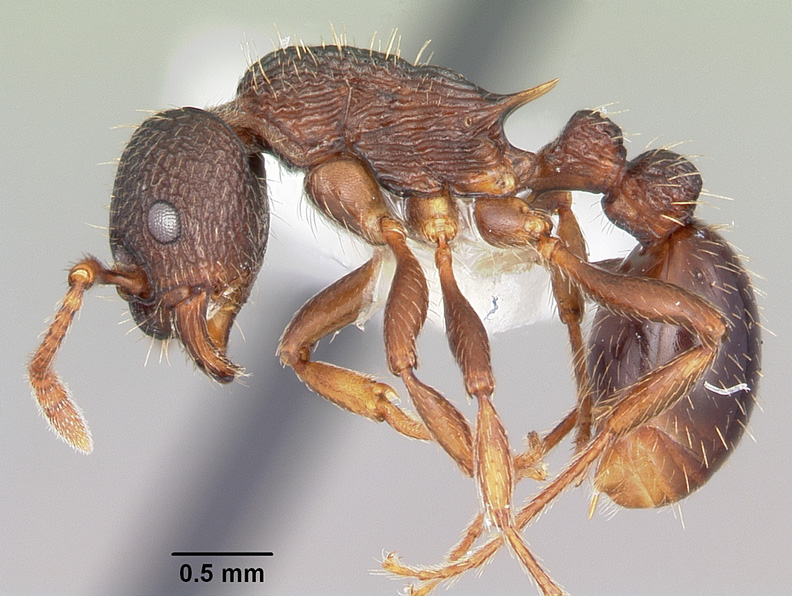This extreme close-up image showcases a brown ant against a gray-blue background, illuminated by a light. The ant's head is facing left, revealing a multifaceted silverish gray eye. Its body, segmented into three parts—head, thorax, and abdomen—is covered in fine, wiry, white hairs. The antennae are particularly notable, extending from the head with even finer hairs. The six spindly, sectioned legs, also adorned with tiny hairs, are visible. In the bottom left corner, the scale is indicated with black text, "0.5 mm," accompanied by a line, providing a sense of the ant's diminutive size.